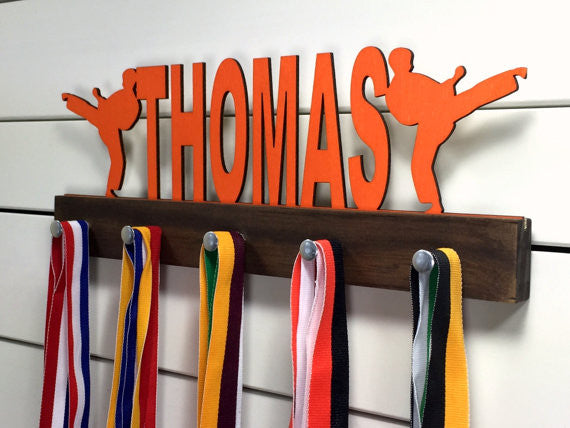The image depicts a wooden coat hook rack mounted on a wall with horizontal white slats interspersed with metal gaps. The rack is oriented at a slight angle, with the foreground on the right appearing closer to the frame than the back left. The dark brown wood of the rack features five evenly spaced, horizontally arranged pegs made of silvery metal. Hanging from each peg are multiple ribbons of various colors, including combinations such as red, white, and blue; blue, yellow, and red; brown, orange, and green; red, white, and black; and yellow, black, and green, though the ribbons are cut off at the bottom, obscuring their full length. Atop the wooden rack, large capital letters spell out the name "THOMAS" in bright orange, flanked by two cutout figures of humans in karate poses, suggesting that the ribbons might be associated with karate achievements. The entire setup is mounted securely to the wall, giving it a functional and decorative appearance.